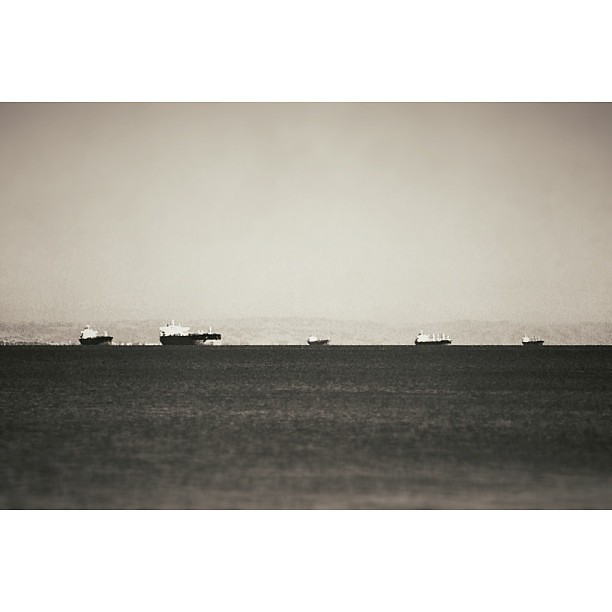This black and white photograph, taken from a boat on the ocean's surface, captures a wide-angle view of a vast cove. The image is marked by a dark, rippling ocean under an overcast, gray sky, with faint outlines of distant mountains on the horizon. Scattered across the water are five large tanker ships, each distinct yet uniformly featuring dark hulls with white superstructures. These tankers, which seem to be anchored rather than moving, are spaced at various points along the cove. The overall ambiance of the scene suggests a somewhat vintage appearance, with the murky water and the sky temporarily merging to frame the stately, evenly spread vessels.